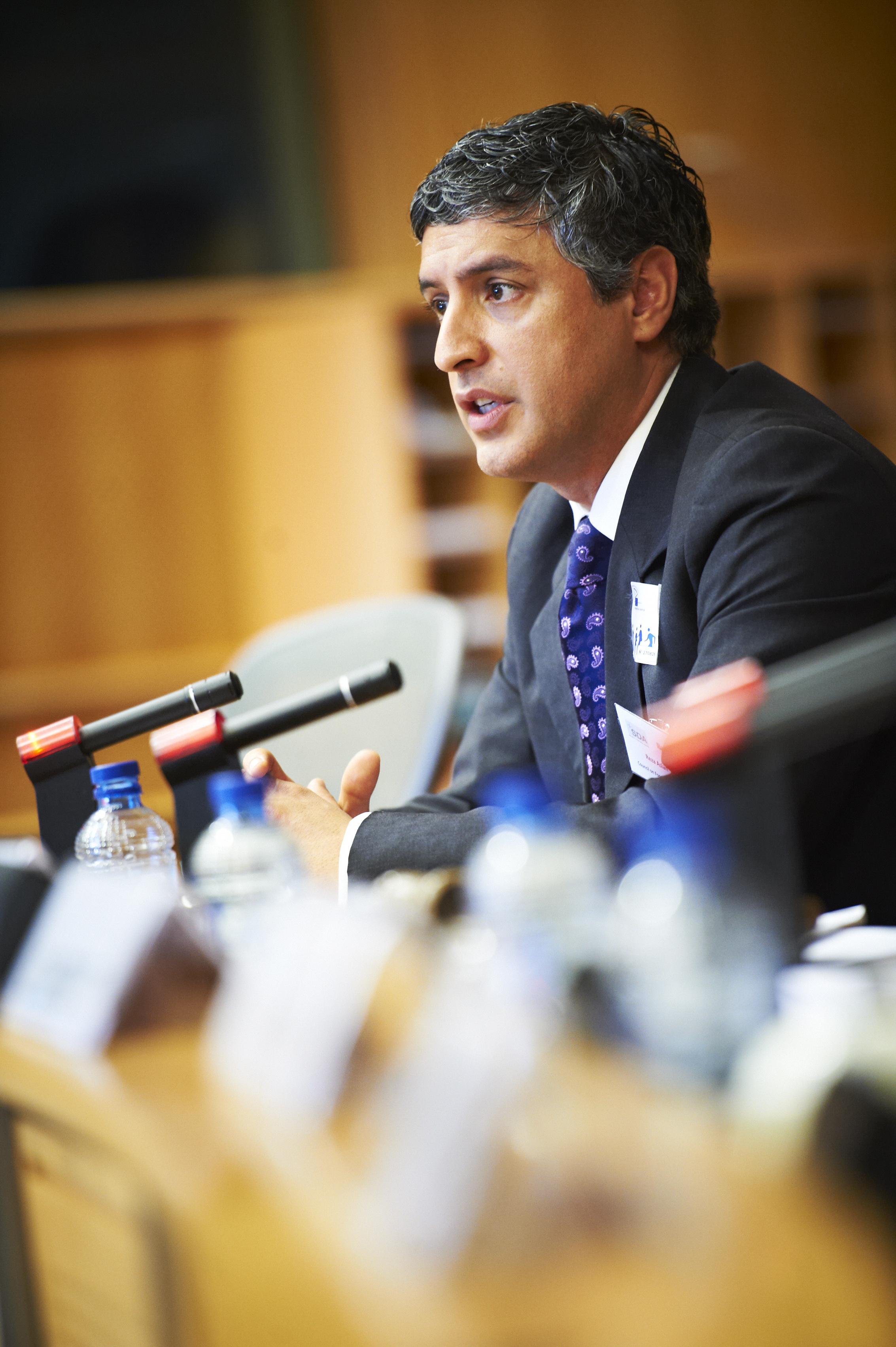The image depicts an official, possibly in his late 40s or early 50s, seated at a wooden desk during what appears to be a press or news conference. The man, whose ethnicity could be white, Hispanic, or Indian, has short, black, greying hair and is dressed in a black suit jacket, white dress shirt, and blue tie. Positioned behind two visible microphones, he is gazing towards the left side of the frame. In front of him, a number of unreadable name tags suggest the presence of additional participants at the table. The background consists of wooden walls, possibly adorned with a black flat-screen TV and a shelf. The table is cluttered with microphones, water bottles, and pieces of paper, likely indicating the identities of the speakers, reinforcing the formal and official nature of the setting. An empty chair sits beside the man, emphasizing the structured arrangement typical of a panel or political meeting.